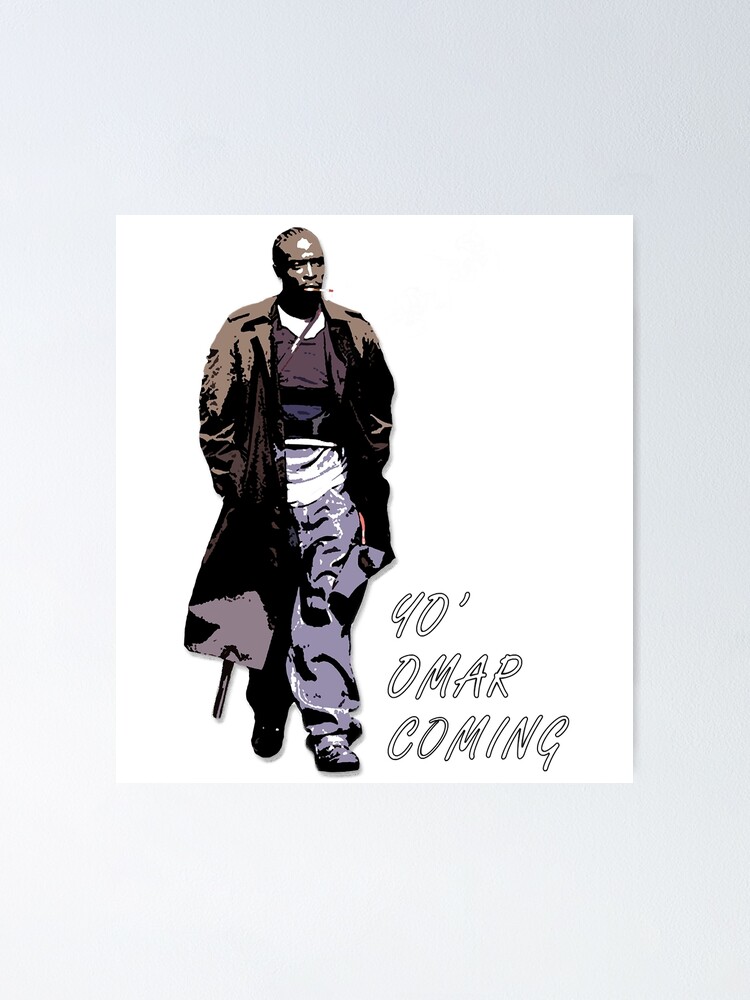The image is a square graphic displayed on a light gray background. The central focus is a stylized, cartoonish black-and-white illustration of Omar Little, a character from the TV show "The Wire," portrayed by the late Michael K. Williams. The illustration captures Omar as an African American man with braids, wearing a long brown trench coat over baggy pants and a T-shirt, with his hands tucked into the pockets of his coat. A strap, possibly for a bulletproof vest or a weapon, runs across his chest, with the barrel of a shotgun subtly protruding from beneath the trench coat. The image employs a stark contrast of shadows and light, adding a dramatic effect. At the bottom right corner of the graphic, white text with a black outline reads, "40 Omar Cumming."